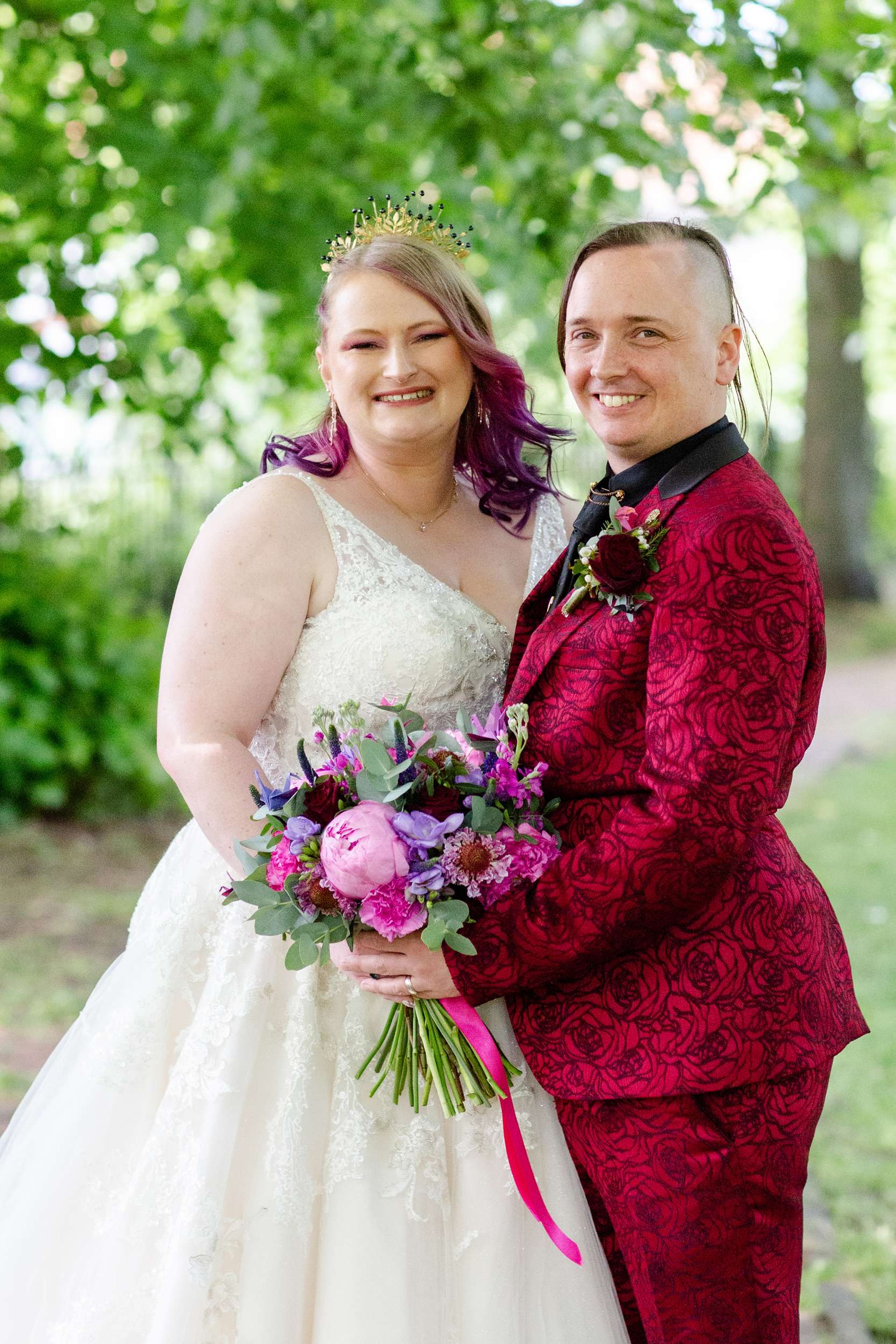This image depicts an outdoor wedding scene featuring a joyful couple standing on a grassy lawn with a backdrop of slightly blurred trees. The bride, a heavy-set white woman with blonde hair transitioning to purple at the bottom, is adorned with a gold tiara with dark-colored gems, gold dangly earrings, and a white, sleeveless, lace wedding dress with a V-neck. She holds a bouquet of pink, purple, and green flowers, shared with her partner, who could be either an androgynous-looking woman or a trans man. The partner's distinctive hairstyle includes a shaved side and slicked-back brown hair. They wear a deep burgundy, rose-patterned suit accented with a dark red rose boutonniere. Both are smiling and looking directly at the camera, sharing a celebratory moment on their special day.